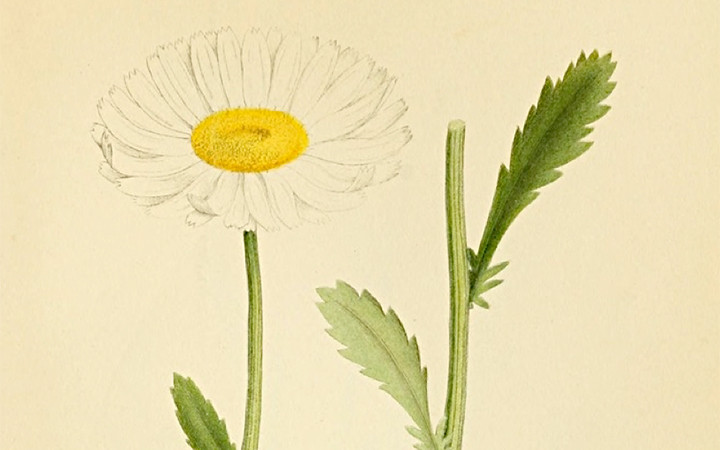This image is a detailed drawing of a flower, specifically resembling a daisy-like dandelion, set against a cream beige background. The primary flower is depicted with white, circular petals encircling a yellowish-orange center. It stands on a green stem with a jagged, pointy green leaf at its base. Adjacent to it on the right is another green stem, featuring two similar jagged leaves, but the flower at its top appears to have been snipped off. The drawing shows meticulous shading and coloration, likely achieved with colored pencils or paint, capturing the natural texture and form of the elements. The scene is straightforward, displaying just the two stems, and the background paper provides a soft, off-white contrast.